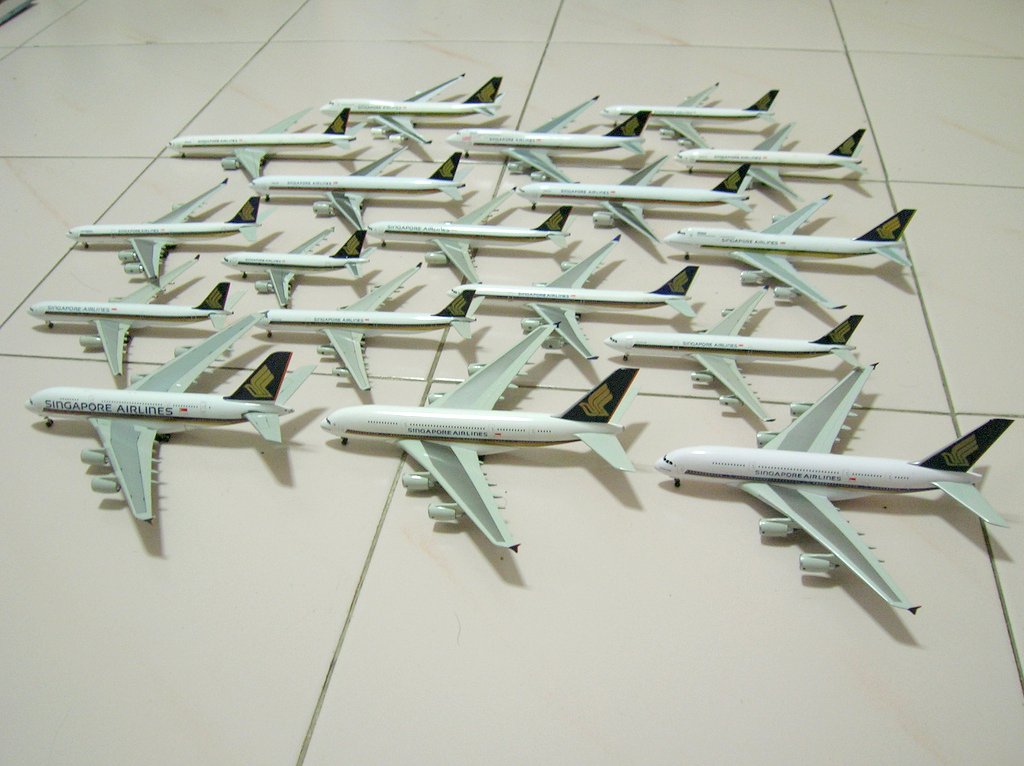The photograph captures a collection of 18 model jumbo jet aeroplanes, arranged in a neat formation of seven rows. The rows on the bottom consist of three planes each, and the rest alternate between two and three planes. All model planes are meticulously aligned horizontally, with their noses, cockpits, and front landing gears pointed to the left, and their tails to the right. They are uniformly designed, showcasing a white fuselage that bears the "Singapore Airlines" logo. The wings, emerging at a slight backward angle, display a greenish-gray color complemented by a darker, uneven stripe that tapers towards the tip. Each wing accommodates two engines. The tail fins of these planes are distinctively navy blue, adorned with a yellow logo. The models rest on a white-tiled floor with dark grout, adding contrast to the overall image.